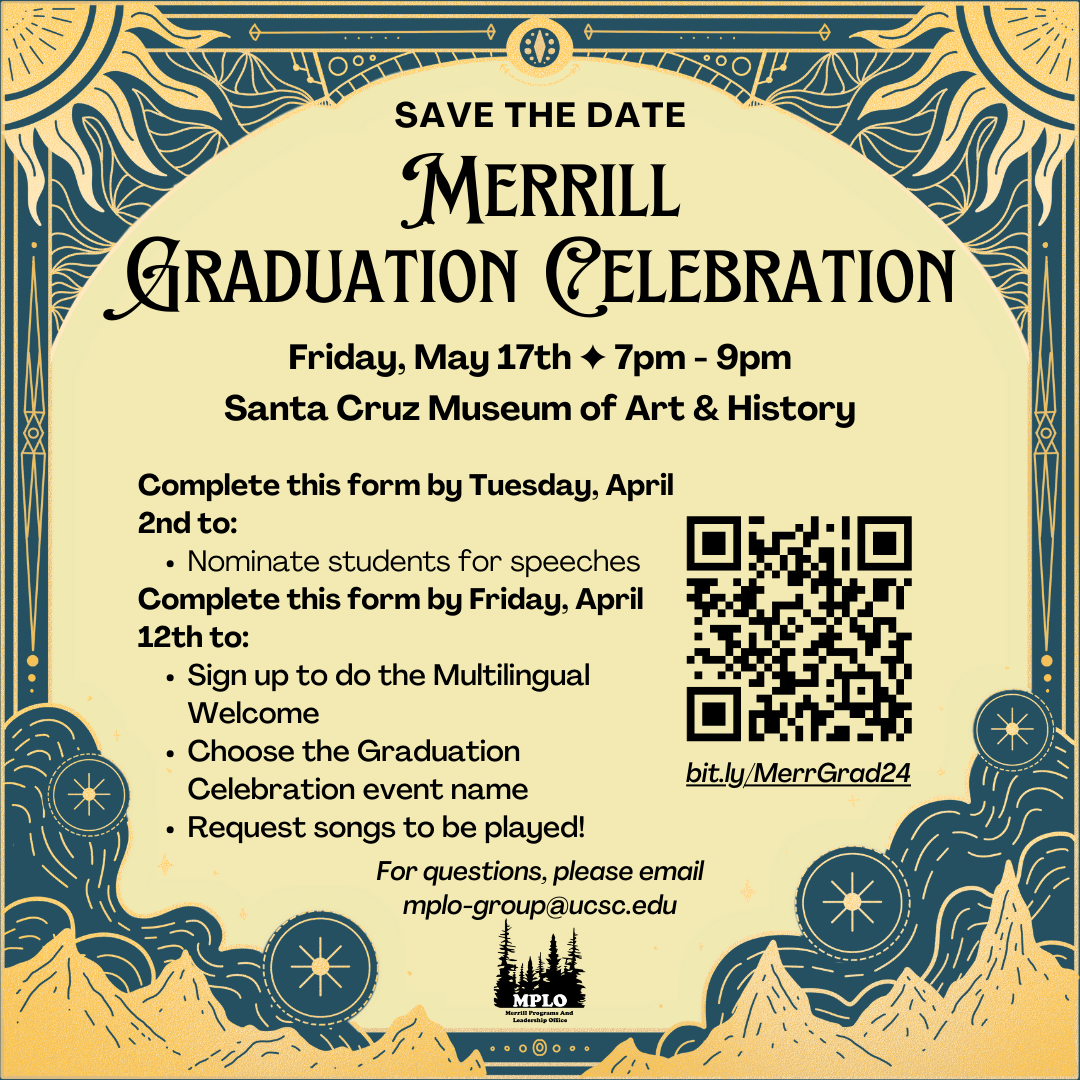This detailed and aesthetically pleasing save-the-date card for a graduation celebration is square in shape. The background is a mix of medium to darkish blue hues and a soft muted yellow. In the upper left and right corners, there are illustrated yellow suns with flame-like rays emanating from them. The bottom left and right corners feature muted yellow mountain ranges. Above these, swirling blue shapes intertwined with yellow lines create an intricate design.

At the center of the card, the main background is a soft muted yellow color. The text at the top is in black font and reads, "Save the Date." Below this, in larger, all-caps, stylized font, it says "MERRILL." Further down, it announces "Graduation Celebration" in a more formal font. The event details are as follows: "Friday, May 17th, 7 p.m. to 9 p.m., Santa Cruz Museum of Art and History," which spans two lines.

On the left side of the card, there is additional text providing instructions to complete a form by Tuesday, April 2nd. It includes several bullet points for details. The right side features a separate column with a scannable QR code beneath which there's a shortened URL reading, "bit.ly/MERRILLgrad24." At the bottom, a courteous "Thank you" is included.